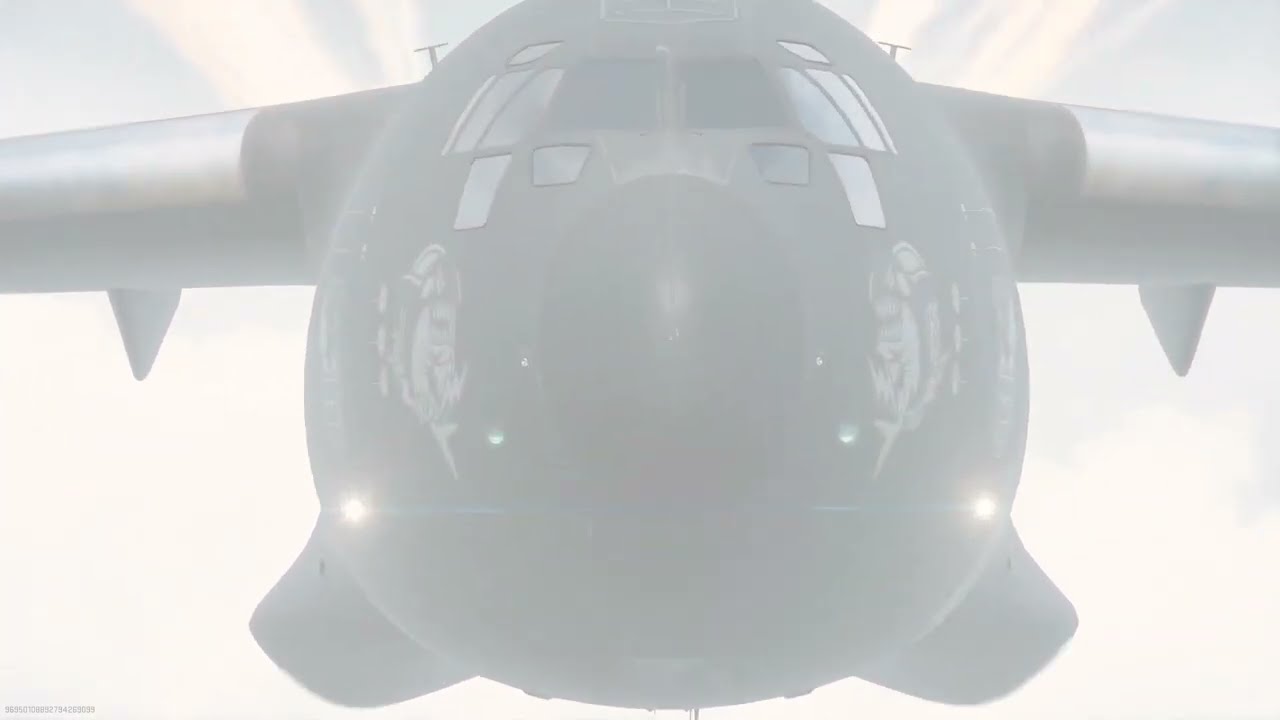The black and white image captures a close-up of the nose of an aircraft, which appears to be coming directly towards the viewer. The photograph, taken through a foggy or smoky lens, shows a highly reflective plane with an egg-shaped middle and two wings extending out of the frame to the left and right. The hazy background displays a uniform mix of light blue and white, enhancing the image's ethereal quality. Reflections of bright lights can be observed over the plane's wings, and indistinct shapes are mirrored on the front of the cockpit, which is otherwise obscured by the light. The wings feature small triangles at their base, and there are two small T-shaped protrusions on each side of the cockpit. Beneath the windows, which are numerous and likely part of a non-commercial, possibly military aircraft, the details become less clear and blend into the enigmatic fog enveloping the scene.